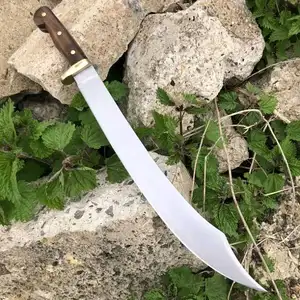This photograph vividly captures a long, curved knife, reminiscent of a pirate's weapon or an ornate dagger, resting atop large, broken concrete boulders. The knife features a brown handle with divots or screws spaced along its length and its silvery blade glistens in the bright sunlight. The knife is centrally positioned, angled with the handle towards the top and the blade extending downwards to the bottom right corner of the image. The background is dominated by green, leafy ground-covering plants that weave and spread between the white concrete fragments, overtaking the rugged terrain. The style of the image is highly realistic, with no accompanying text to explain the context, leaving viewers to ponder the scene's story and reason.